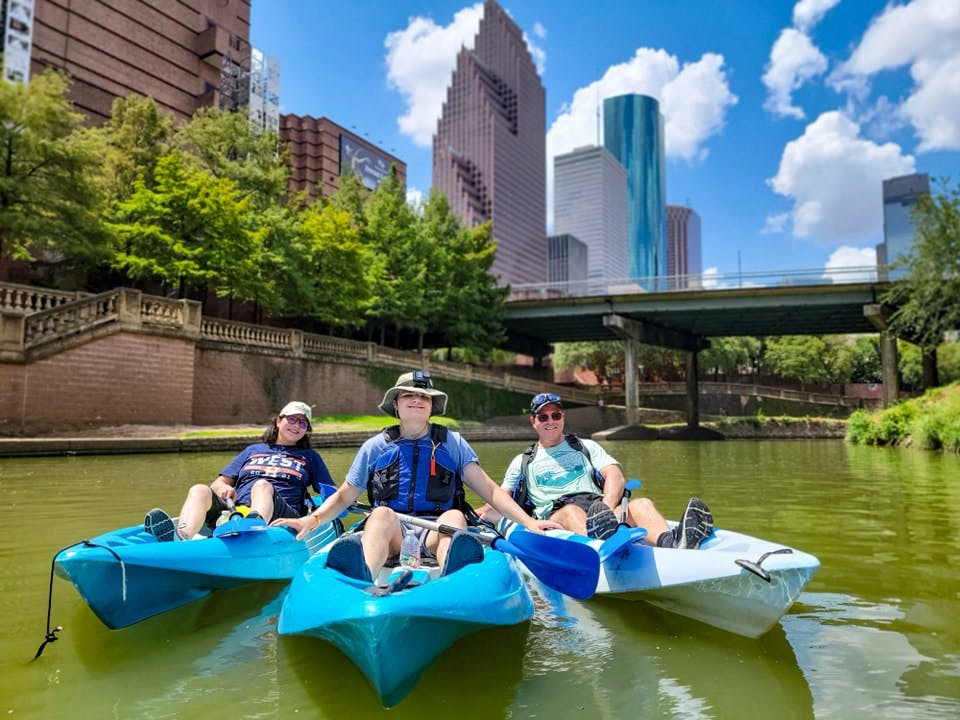In this vibrant photograph, three people are kayaking on a greenish-colored river in the midst of a bustling city. Captured from a front-facing perspective, the three kayakers are positioned close together, smiling directly at the camera. The person in the middle, who has a brown floppy hat, joyfully holds onto the kayaks of the individuals on either side. To the left, a person who presents as female is seen wearing a blue shirt with writing, glasses, and a hat, and paddling a bright blue kayak. On the right, a slightly chunky man with sunglasses, a blue hat, and a light blue shirt is in a white kayak. The river is framed by lush greenery, with trees and plants visible on both banks, and an array of towering skyscrapers and a bridge or overpass providing an urban backdrop. The blue sky, adorned with fluffy white clouds, adds a touch of serenity to the lively cityscape.